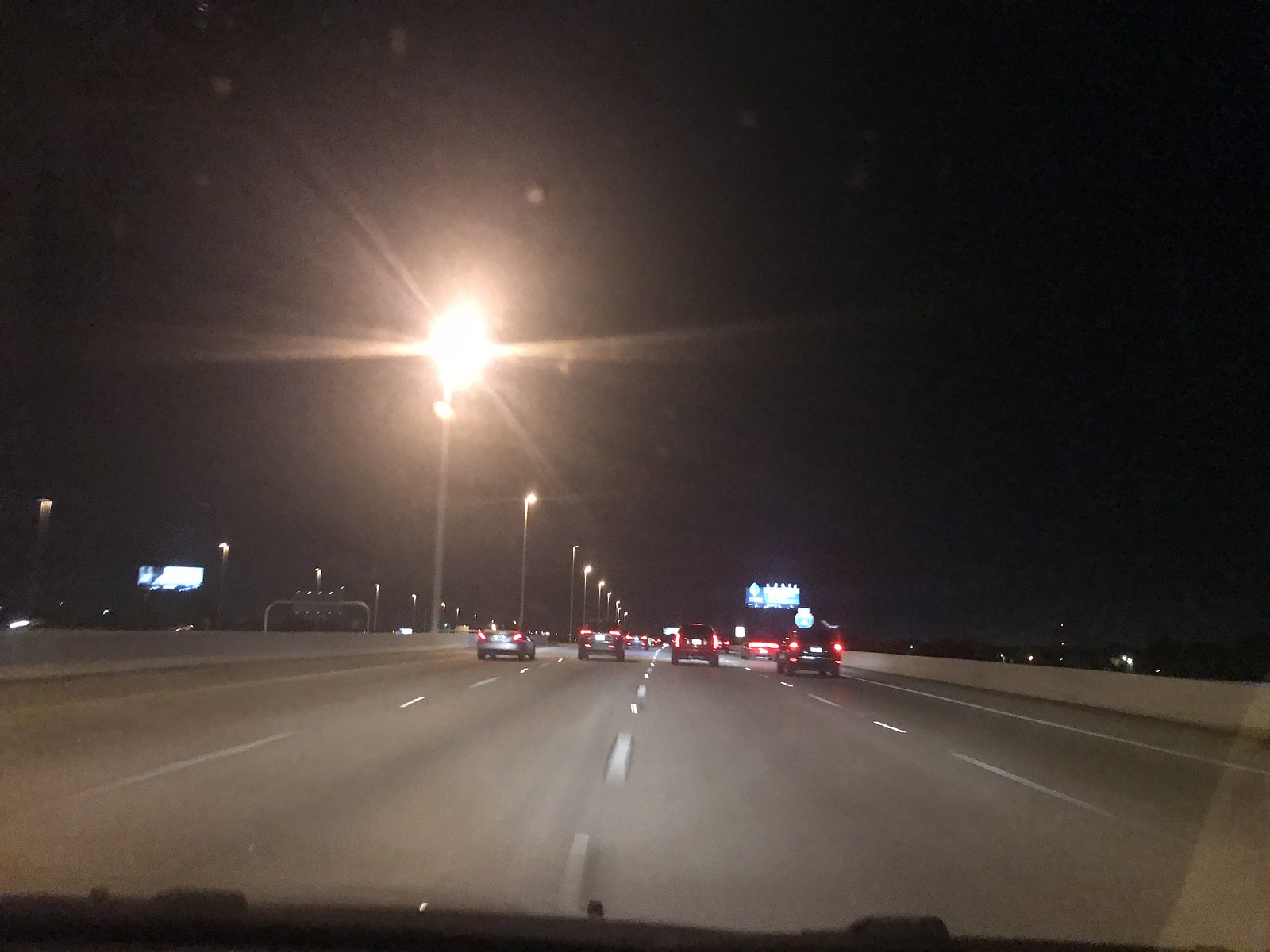Captured from the driver's seat of a car during nighttime, this image provides a detailed glimpse of a bustling four-lane freeway. Numerous vehicles populate the road, their headlights creating streaks of light as they move. A row of street lamps positioned along the central median illuminates the scene with a steady glow. On the far right, a green freeway sign, brightly illuminated, is visible, though its details remain indistinguishable due to its distance from the camera. The overall atmosphere conveys the relentless activity and energy of nighttime urban traffic.